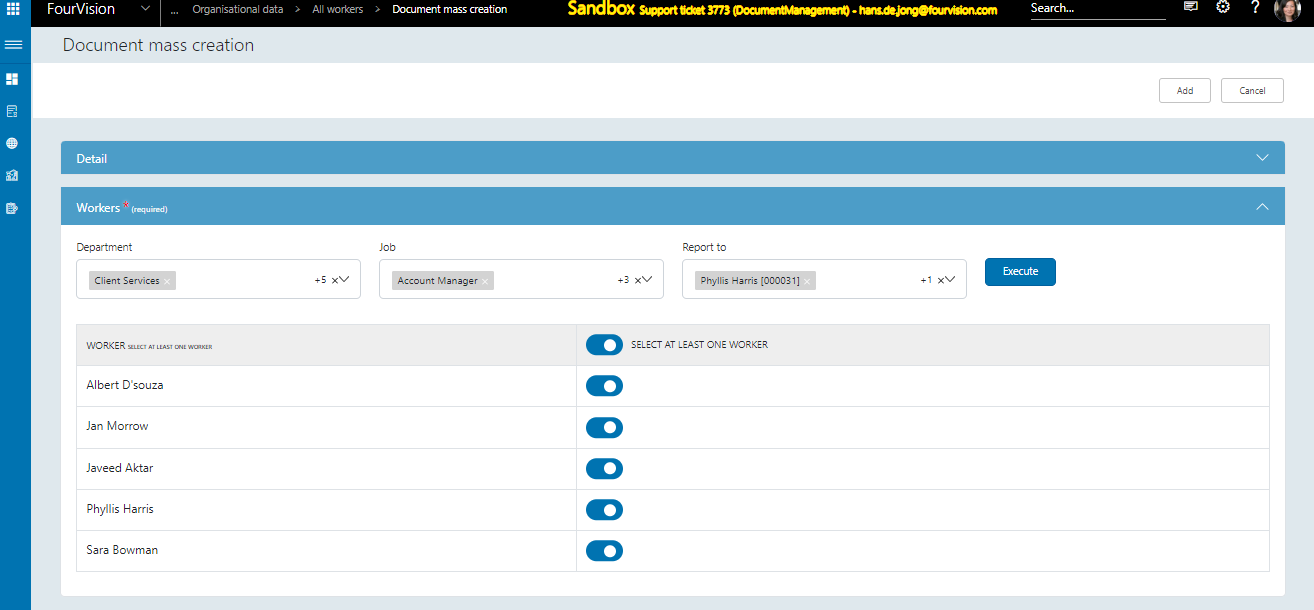This screenshot captures a user interface from a platform labeled "4-Vision," as indicated by the small text at the top. On the upper left corner, within a vertical blue bar, there are several icons, though their specifics are unclear. Next to "4-Vision," there is some text in yellow font mentioning "Sandbox supports..." followed by text too small to discern, and there is a search button nearby. To the right, one can see profile pictures and additional icons.

Below this area, the header "Document Mass Creation" is prominently displayed, accompanied by a long white space and "Add" and "Cancel" buttons on the right. Beneath this section, there's a blue bar labeled "Detail" with a downward-pointing arrow, followed by a section titled "Workers." An upward-pointing arrow appears alongside the header.

Further down, another blue bar titled "Department" is visible, along with likely subsections labeled "Jobs" and "Report To," although the text is very small and hard to read. Each subsection features fields filled with text boxes and various arrows. To the right of the third subsection is an "Execute" button of unspecified function.

At the lower part of the screenshot, a list is shown with a slider button next to each item. All sliders are blue, indicating they are turned on. The top line of the list states "Select at least one worker" next to the label "Worker." Below this, a series of names presumably identifies workers, but the text is too small to read clearly. Each worker's name is accompanied by a blue slider button, all in the active position.